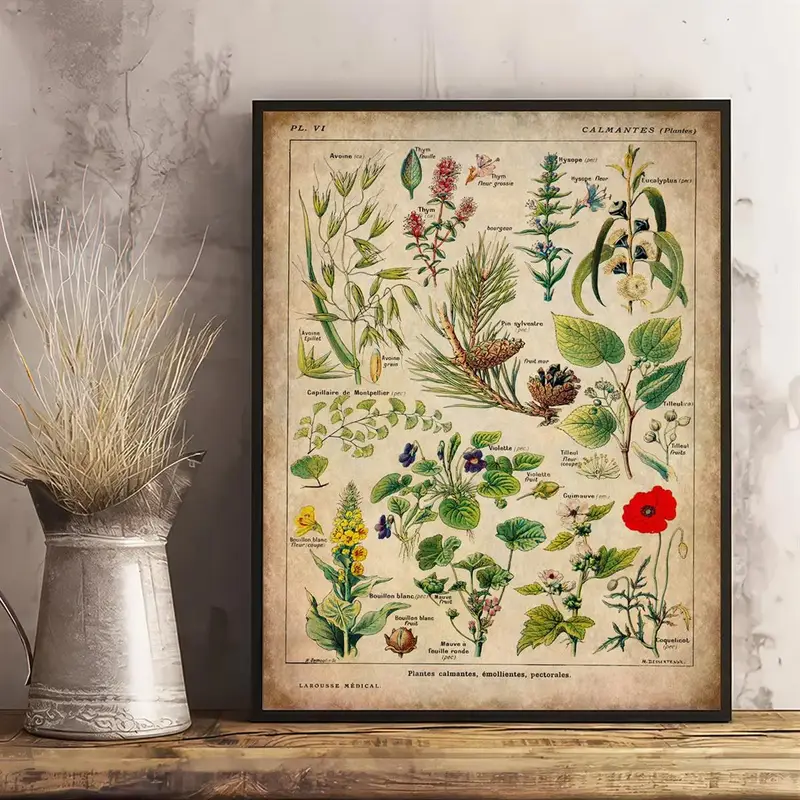The image depicts a framed vintage botanical illustration set on a rustic wooden countertop. The black frame encases several detailed depictions of plants, each labeled with scientific names and descriptions. The upper left corner features the text "PLV1," while the upper right reads "Calmantes" followed by an illegible word in parentheses. Dominating the center is a pine tree segment, showcasing needles and pine cones. Surrounding this centerpiece, the illustration includes a vine with green leaves and purple flowers above it, and a plant with frayed buds in the top left corner. To the right, a plant bears red flowers, and in the upper right corner, there's a plant with white flowers and long, thin leaves. Below this, a plant with small green leaves and berries can be seen. Further down, a red poppy-like flower is depicted, adjacent to a blackberry vine-esque plant with small white blossoms. Completing the botanical ensemble in the bottom left corner is a plant with yellow flowers. To the left of the framed illustration sits an old-fashioned silver pitcher with intricate floral designs, filled with tall grasses. The entire setup is against a wall with distressed tan wallpaper, adding to the image's vintage farmhouse aesthetic.